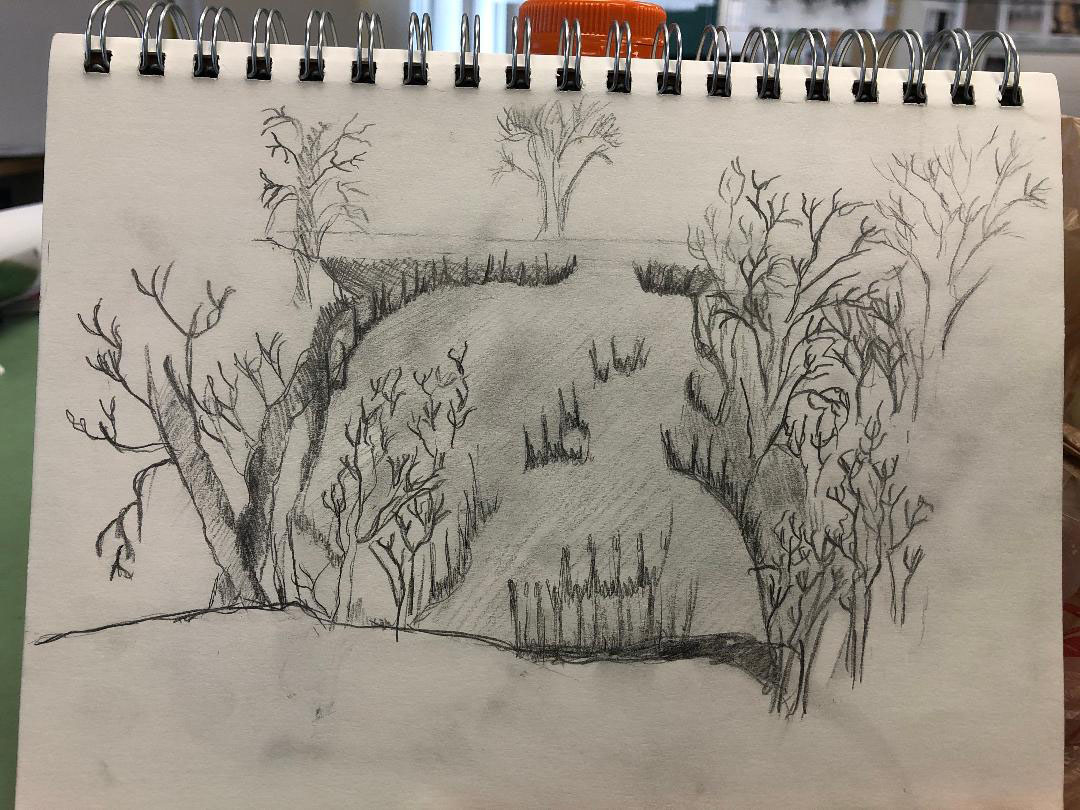The photograph captures a detailed pencil sketch on a white sheet of German notepad paper, bound by visible silver spiral rings at the top. The pencil drawing illustrates a rectangular field surrounded by mature trees with numerous branches but no leaves, suggesting a winter scene. The field features varied grass lengths, with some areas having taller marsh-like grasses or reeds. The sketch includes a possible fence in front of the trees, adding depth to the landscape. In the background of the photograph, beyond the notebook, there is an orange cap, a white wall, and some windows, indicating an indoor setting. The edges of the paper show gray smudging, particularly at the bottom and on the right side, adding a weathered look to the drawing.